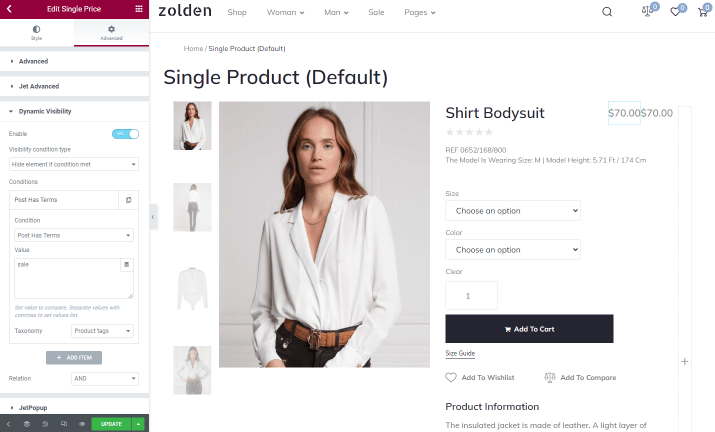The image is a screenshot from an e-commerce website named Zoldin. The page appears to be showcasing a product, specifically a white V-neck shirt and bodysuit combination. 

On the left side of the screen, there is a wide column featuring various toggle switches, search boxes, and selection options; however, the text is not clearly readable. 

The top of the right side prominently displays the Zoldin logo, followed by several category options: Shop, Woman, Man, Sale, and Pages. In the upper right corner, there are icons representing a shopping cart, which likely offers quick access to the cart, express list, and possibly other account features. There's also a search bar with a search icon.

The main part of the image highlights a product page with a large photo of a slim woman with long hair, modeling the white shirt and bodysuit. The garment is distinguished by its V-neck, long sleeves, and a jean puffer accessory. Below this main image, there are several smaller thumbnail images showing different views of the product. One thumbnail displays a view of the garment on its own.

To the right of the photos is a detailed description of the product. The item is priced at $70 and includes information such as an item number. There's also a drop-down menu for selecting sizes and colors. Another menu allows the user to choose the quantity they wish to purchase. Further below, there is a section for product information, which is partially cropped off but contains details about the V-neck.

Overall, the page is typical of what one might find on any e-commerce platform, offering thorough details and multiple viewing options of the product to assist in the purchasing decision.